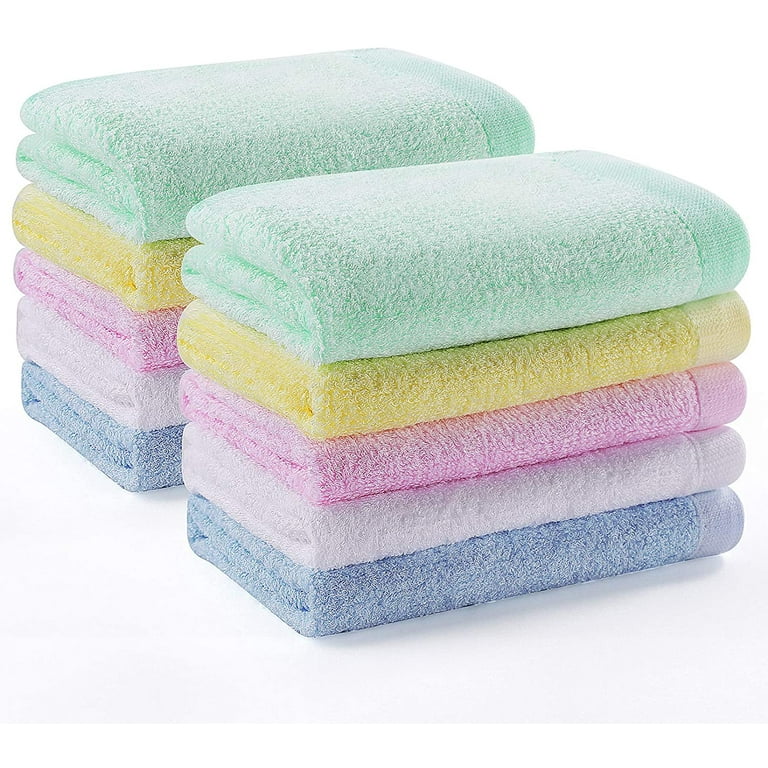This photograph captures an assortment of neatly folded pastel bath towels arranged in two symmetrical stacks of five on a plain white background. Each towel is carefully folded into a precise rectangular shape, ensuring both stacks are identical in dimensions. Viewed from an angled perspective, the edges of the towels create a visually appealing symmetry. The front stack displays all its details prominently, while the back stack is visible at an angle, with just the edges peeking out. Both stacks follow the same color sequence: the bottom towel is a deep blue, followed by a very light bluish-white, a pinkish middle towel, a yellow one, and topped with a teal or light green towel. Each plush towel is accented with a thin strip along the edges, emphasizing their softness and quality.